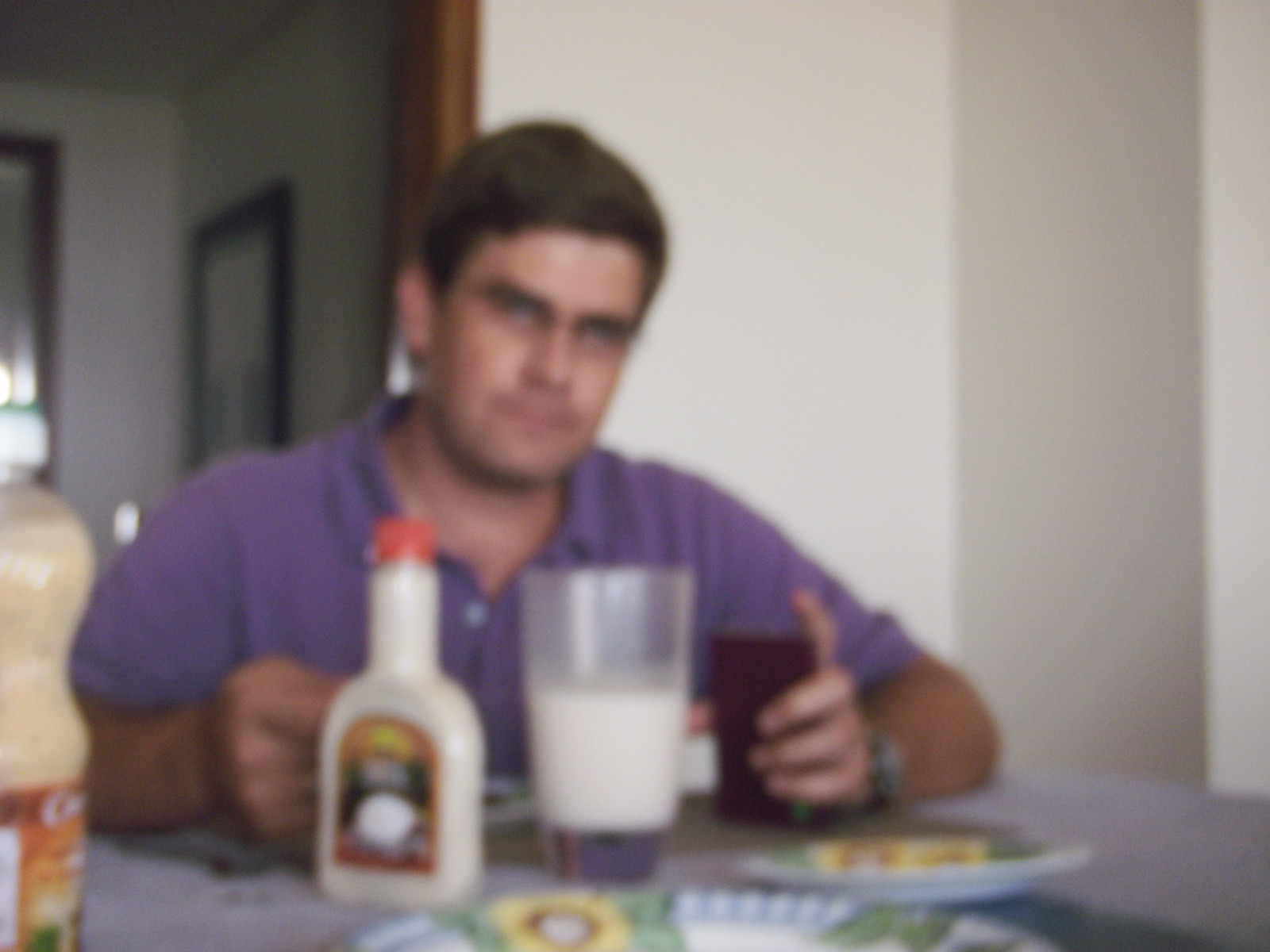A man with short dark hair and caramel-colored skin, possibly of Asian or Hispanic descent, is seated at a dining room table in a well-lit indoor setting. The room behind him is empty, featuring a stark contrast of dark shadows against white walls. The man, with thick dark brown eyebrows, has a neutral expression on his face, although the photograph is slightly blurred. He is holding a dark brown plastic tumbler in his right hand, with the contents of the glass unclear, possibly a beverage or water. In front of him, there is a clear white glass, half-filled with milk. To the left of this glass stands a bottle of white salad dressing, its exact variety not identifiable. The man is dressed in a short-sleeved, purple polo shirt, with both of his elbows bent and hands resting on the table. A white plate of food, the contents of which are not decipherable, is placed in front of him, along with other indistinguishable items on the table.